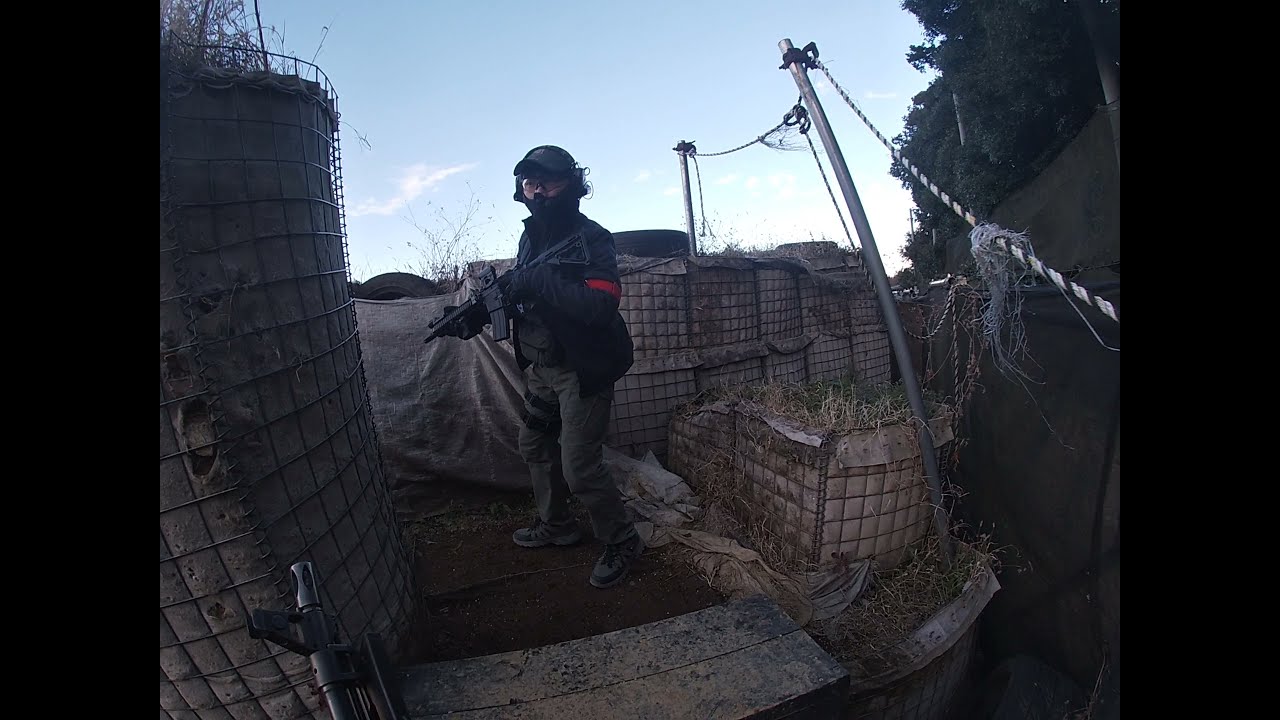In the forefront of the image is a man engaged in a paintball match, positioned slightly left of center and looking back at the camera. He is outfitted in protective gear, including a black baseball hat, a face mask with a visor, and a dark winter coat adorned with a red band on the sleeve of his left arm. He wears dark brown pants and is gripping a large, black, automatic-looking paintball gun with both hands, the butt of which rests against his shoulder while the muzzle points to the left. The scene around him is filled with various paintball course obstacles, such as stacked hay bales, metal wiring, and a rope providing additional cover from the right side of the image. In the background, there are elements of the course including a tire used as cover and several trees in the upper right corner. The edges of the photo contain black rectangles, framing the intense, action-packed moment on the paintball field.